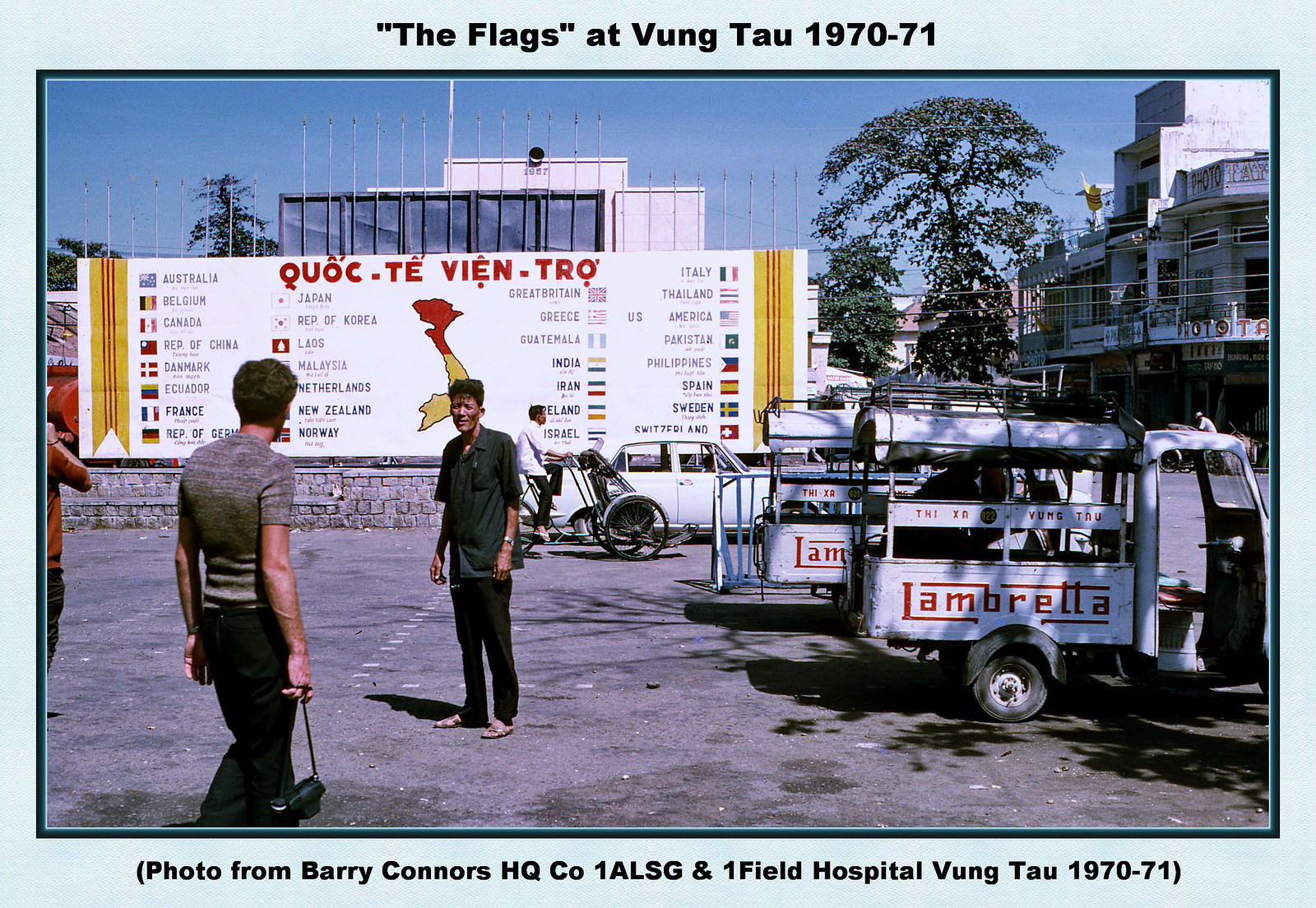This photograph, evidently from the early 1970s in Vietnam, depicts an outdoor street scene, framed with a light blue border that reads "The Flags at Vung Tau 1970-71" at the top and "Photo from Barry Connors, H. James Co., 1 ALSG and 1 Field Hospital, Vung Tau 1970-71" at the bottom. Central to the image, two men face off approximately 10 feet apart, seemingly engaged in a tense interaction. They are both dressed in grayish shirts and dark pants, one holding an object on a chain by his side. Surrounding them, several other people are either standing or moving in the background, including a man riding a bicycle. The scene is set in what appears to be a parking lot with gray pavement, populated by various vehicles including white motor trikes and work trucks bearing the name "Lambretta" in red print. Dominating the background, a large billboard features a map of Vietnam adorned with multiple country flags and text that reads "Kyok Ti Win Tro." This billboard appears to serve a political or informational purpose. On the right side of the photograph, there are low-rise buildings and trees, all under a clear blue sky, suggesting a bustling urban setting in Vung Tau.